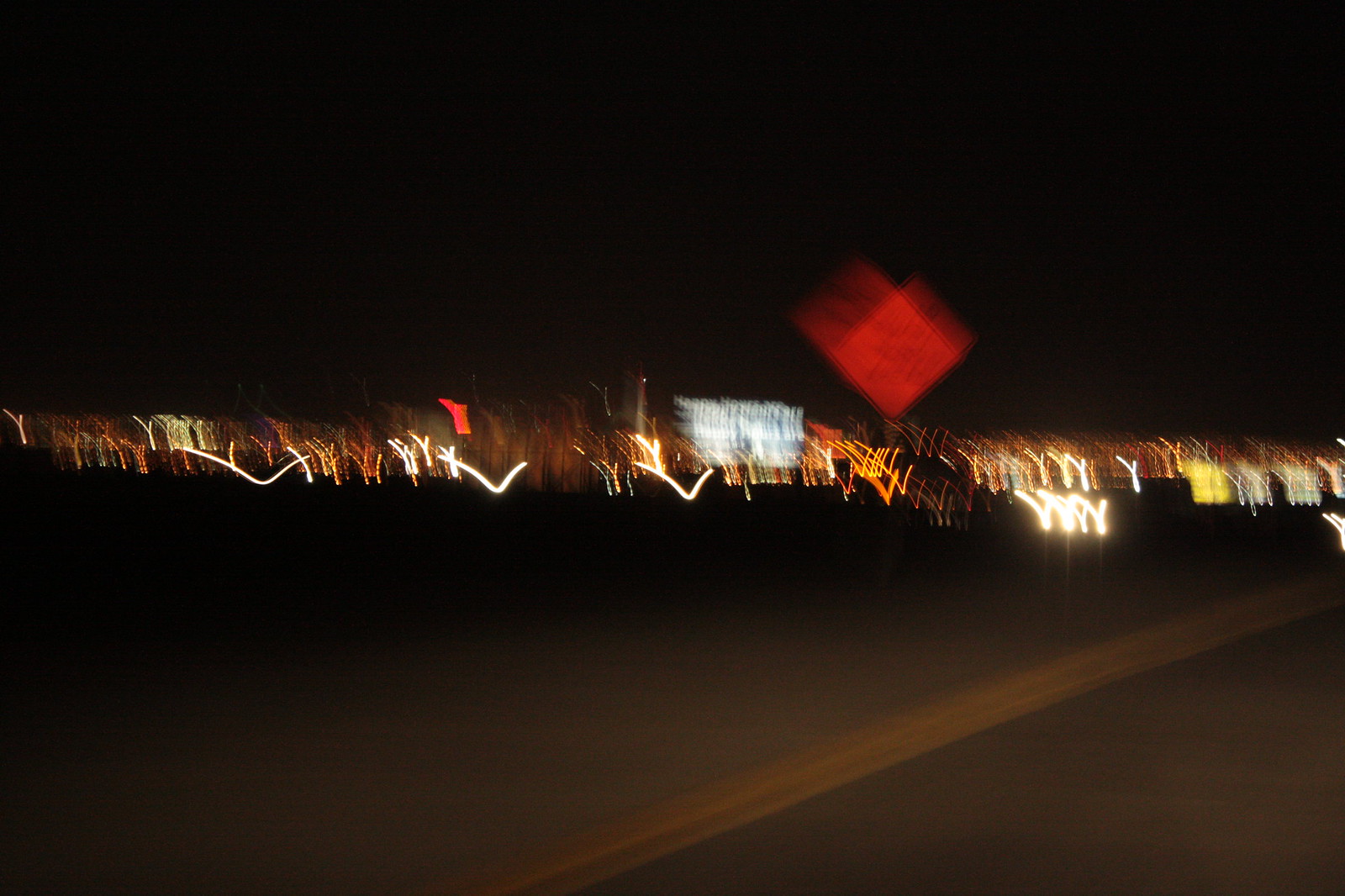This color photograph, taken at night, captures a city skyline with an array of colorful lights—white, yellow, red, and silver-white—blurring into streaks due to motion or time-lapse effect. The foreground features a highway with a visible yellow line running diagonally from the center to the right side, indicating a road divider. Adjacent to this road, there is a diamond-shaped road sign reflecting an orange hue, though the text is unreadable due to the image's blur. The background is dominated by a pitch-black sky, emphasizing the vivid lights and the nighttime setting, creating a stark contrast against the dark surroundings.